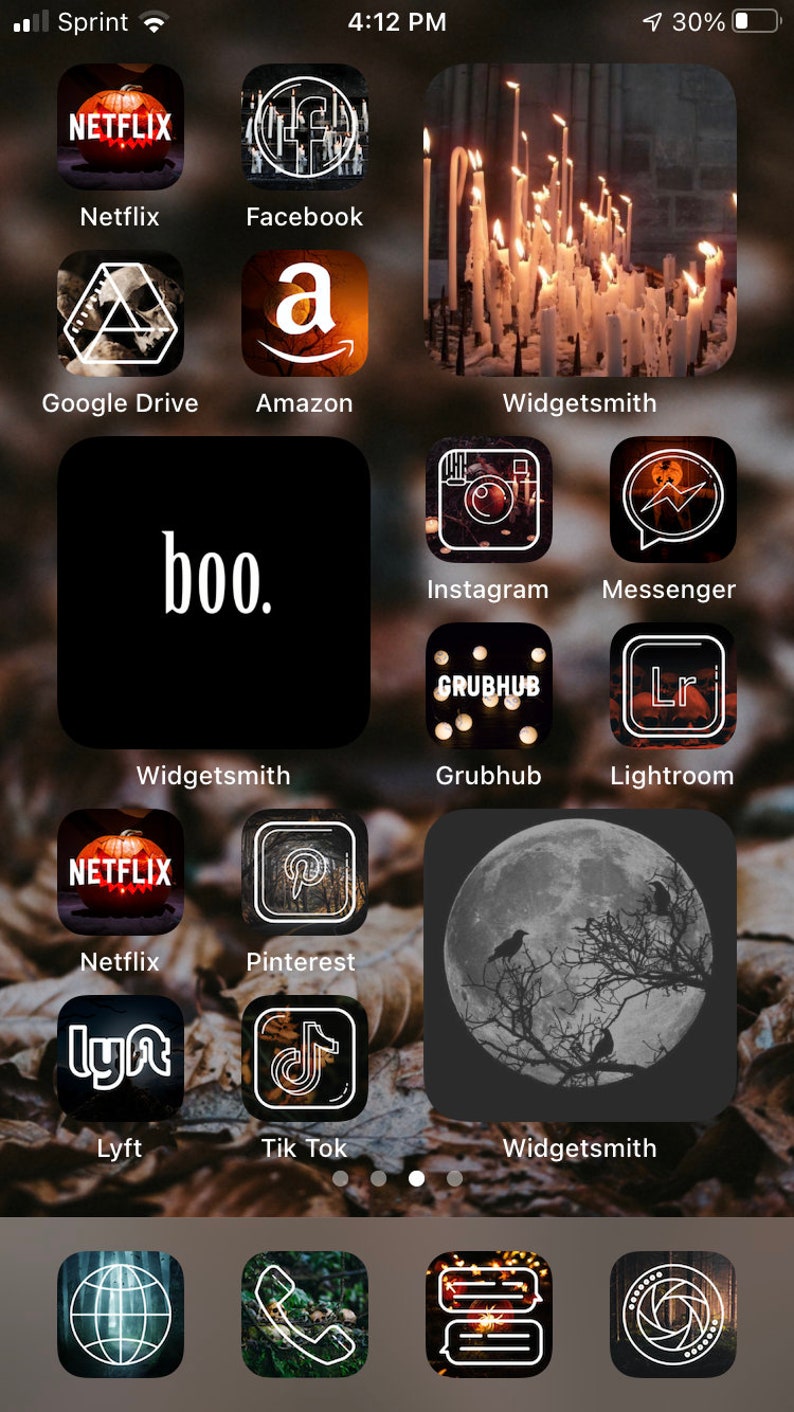The image depicts a smartphone screen displaying a series of app icons against a blurred, possibly autumn-themed background. In the top left corner, two bars indicate the cellular signal strength, followed by the carrier name "Sprint" and a Wi-Fi icon. Centered at the top of the screen is the time "4:12 PM". The top right corner shows an upward arrow with "30%" and a battery icon.

The home screen is organized into rows of app icons. The top row features icons for Netflix and Facebook. The second row displays Google Drive, Amazon, and WidgetSmith. A black WidgetSmith icon with "Boo." written in white is also visible. Additional apps include Instagram, Messenger, GrubHub, Lightroom, another Netflix icon, and Pinterest. Further down, there are icons for Lyft, TikTok, and yet another WidgetSmith widget, this time showing a large globe with a bird perched on bare branches. At the very bottom of the screen, four more icons can be seen, though they are not specified in the description.